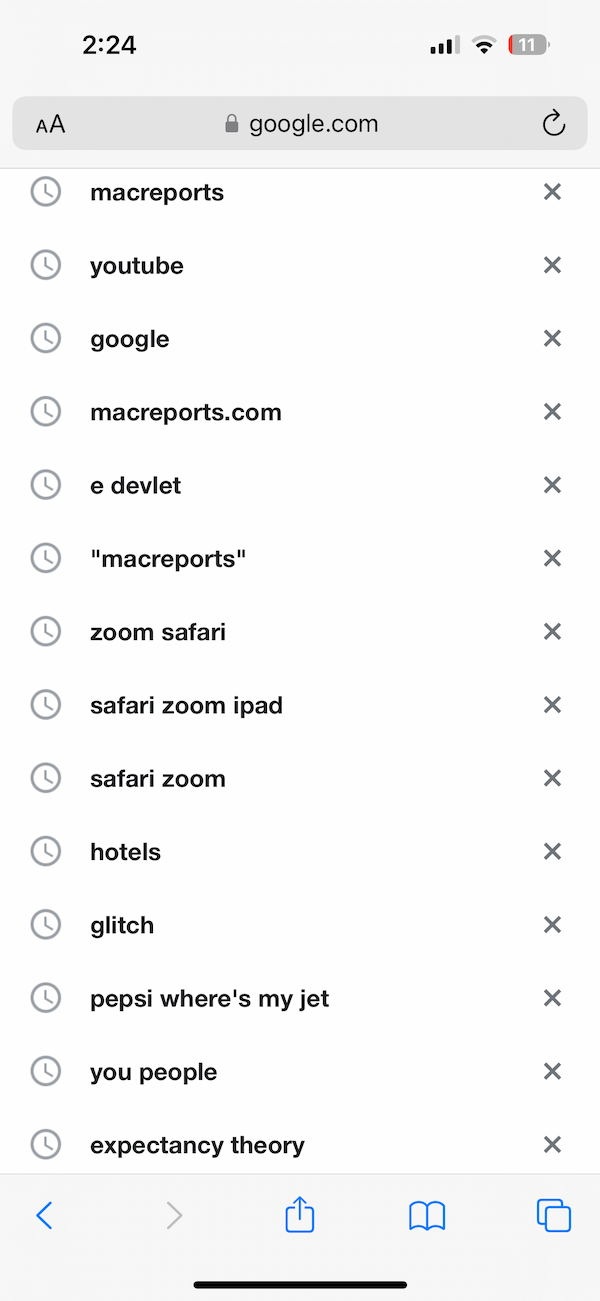This image showcases a cell phone screen with a grayish background. In the top-left corner, the screen displays the time "2:24", while in the top-right corner, three bars indicate the internet service strength and two bars show the Wi-Fi signal. Adjacent is a battery icon, which is only 11% charged.

Below this status bar, there's a Google search bar with the URL "google.com" displayed. Under the search bar is a list of web links, each marked with a small gray clock icon on the left and a tiny "X" on the right. The links are as follows:
1. Mac Reports
2. YouTube
3. Google
4. MacReports.com
5. eDevlet
6. "MacReports"
7. Zoom Safari
8. Safari Zoom iPad
9. Safari Zoom
10. hotels
11. glitch
12. Pepsi Where’s My Jet
13. you people
14. expectancy theory

At the bottom of the screen, there's a standard internet navigation bar with a gray background. It includes a left arrow, a right arrow, a share button, a bookmark icon, and a copy icon. Additionally, at the very bottom of the image, a black line indicates the phone's main navigation bar.